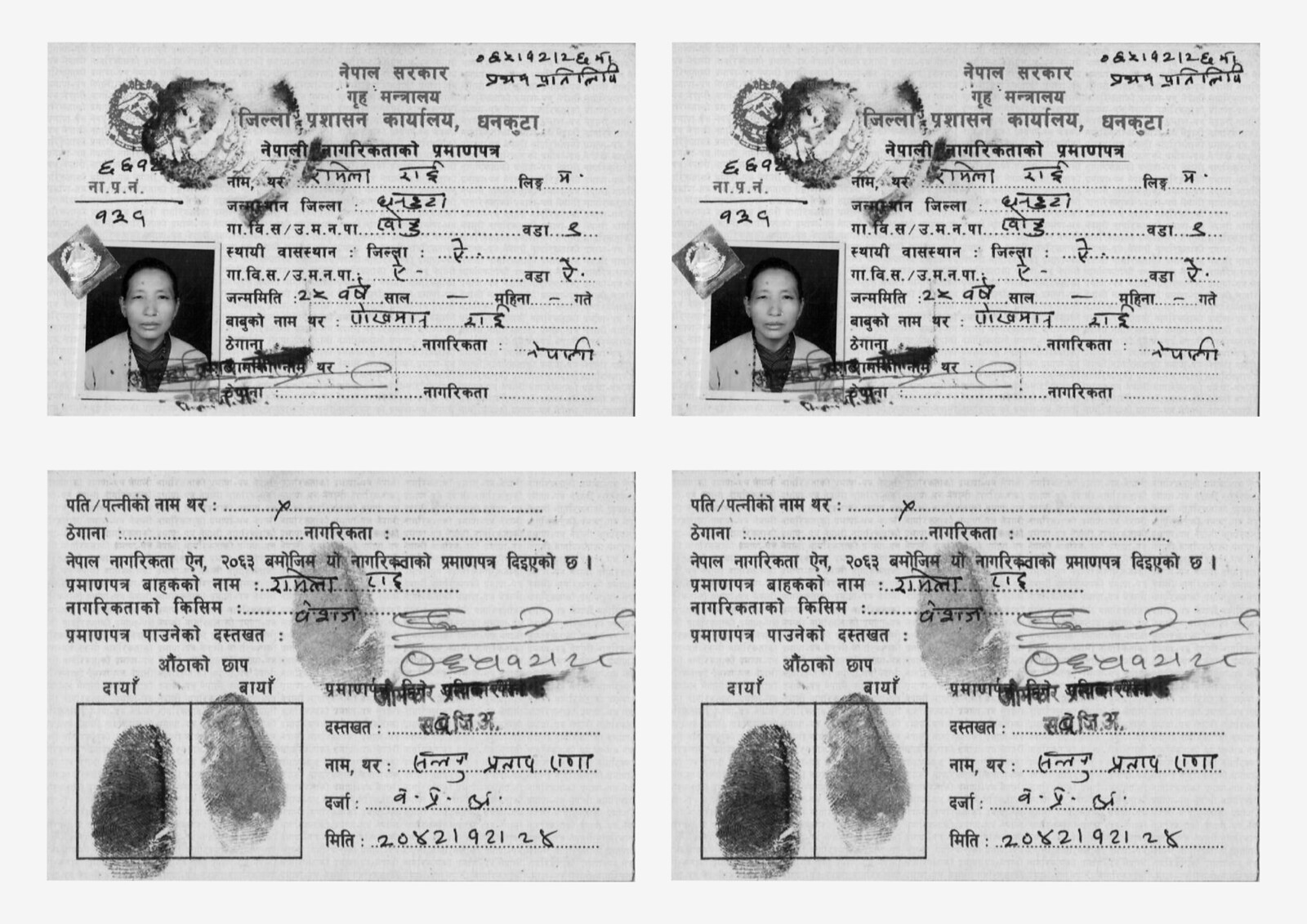The image is a slightly wider than tall, black-and-white photograph displaying two pairs of what appear to be identification documents. Each document features a portrait of the same Asian individual, who appears to be wearing a lab coat, indicating a professional, possibly medical, background. The documents are written in an unidentifiable Asian script, with each document pair consisting of an upper portion containing the portrait and a lower portion showcasing thumbprints, likely from both hands. The identification papers on the right are exact replicas of those on the left. Additionally, the documents contain stamps and watermarks, suggesting official authentication.